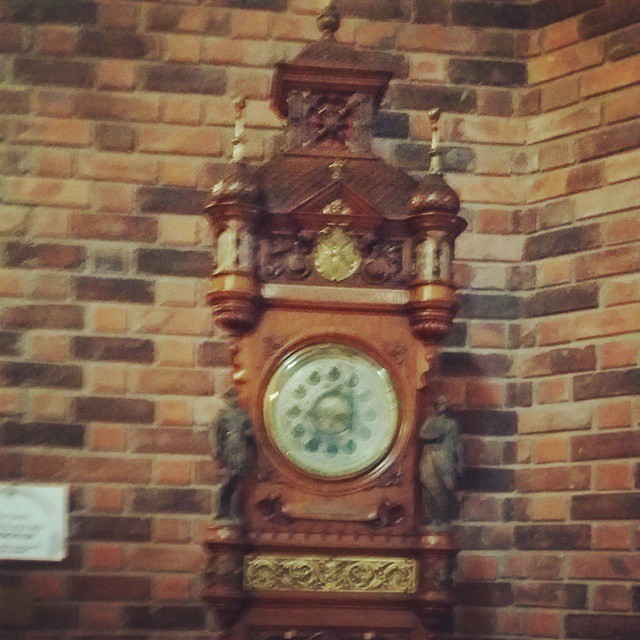This image showcases an ornate antique clock standing majestically against a rustic brick wall. The timepiece, likely hailing from the late Victorian or early Edwardian period, is a testament to exquisite craftsmanship. Its rich woodworking details are vividly on display, featuring intricate carvings and decorative embellishments that add to its historical charm. At its pinnacle, a small peaked roof-like structure is adorned with finials and delicate floral or foliate carvings, enhancing its elegant silhouette. Below, the larger central body houses the clock face, which is meticulously enclosed behind a glass cover. The clock face is surrounded by a frame adorned with Roman numerals marking each hour, though the precise position of the clock hands remains unclear due to the image's slight blurriness. This antique clock, with its elaborate design and historical essence, stands as a beautiful relic from a bygone era.